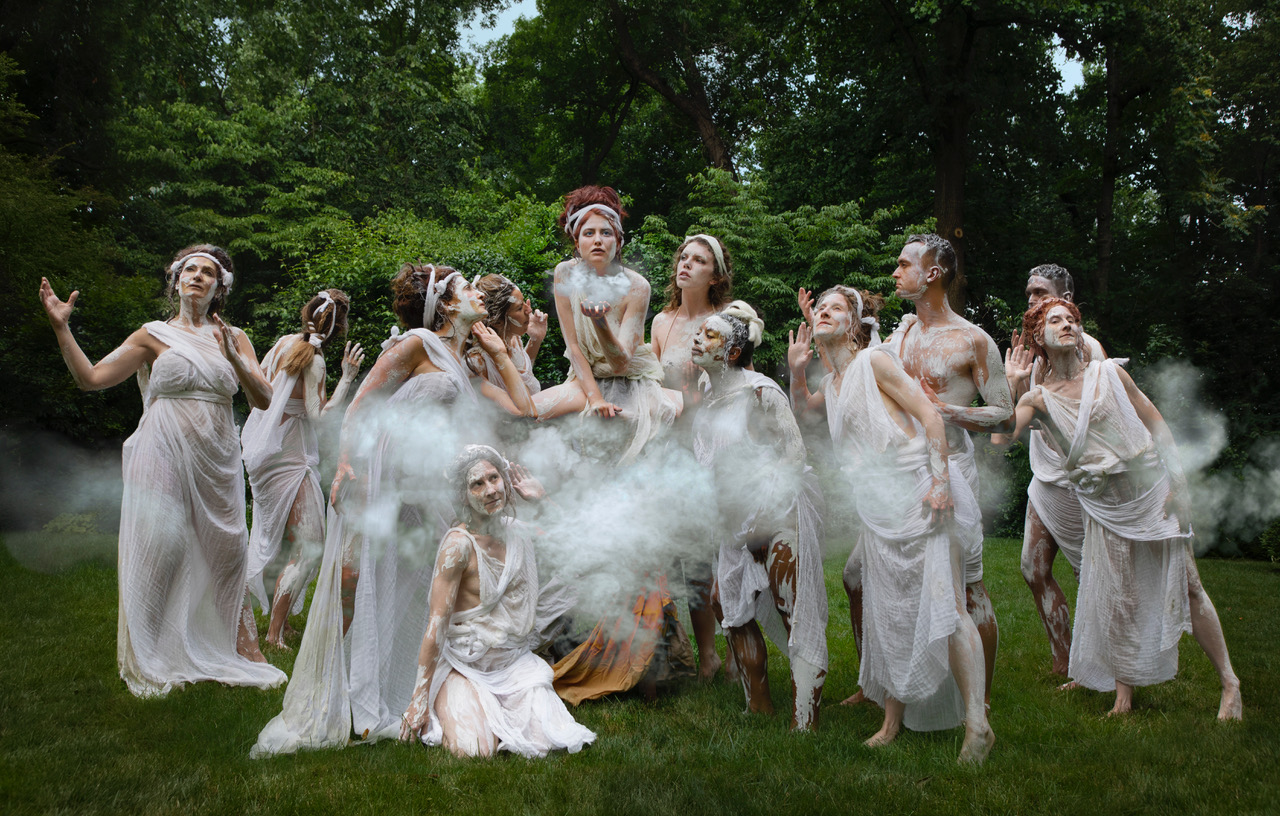This image depicts an ethereal outdoor scene in which a group of about 10 to 12 men and women, dressed in long, white, gauzy outfits reminiscent of togas or shrouds, gather on a lush green lawn. Behind them, a thick wall of trees and bushes stretches up, allowing just a glimpse of blue sky to peek through the foliage. The presence of white smoke or mist adds to the mystical atmosphere. The individuals, including one or two older men and one black woman among mainly white participants, all have parts of their bodies and faces covered in white paint. Many of the women have white ribbons or bands securing their hair, and several members of the group are striking poses with their arms raised—right hand up for those on the left and left hand up for those on the right—suggesting they might be listening to something. One individual appears to be sitting on a large rock with a piece of orange cloth draped over it. Tiny yellow flowers adorn one of the trees, enhancing the vibrant setting, which looks alive and vivid in the daytime light.